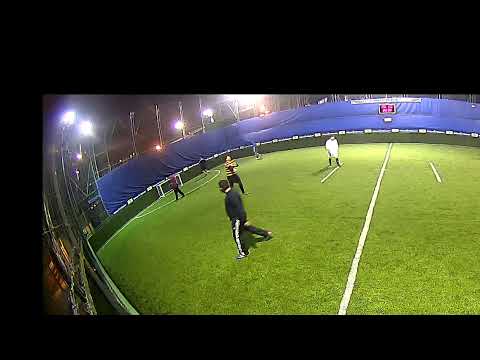The image captures a well-lit soccer field under bright spotlights at night, characterized by its vibrant green grass. Encompassing the field are blue seats, draped in a blue tarp that serves as a makeshift fence. A goal post, with its PVC frame, is positioned towards the left side of the image. The scene includes several individuals scattered around the field, engaging in various activities. In the foreground, a man dressed in a black track suit with a white stripe down the pants walks to the left. Additional figures include a person in a black and yellow t-shirt with black pants, another in a white t-shirt and shorts, and others who are less distinct but visible near the goal post, including one in a red shirt and another in black shorts. The white lines marking the field further emphasize its purpose. Although there is no ball present, the scene is set against a pitch-black sky, highlighting the bright illumination of the overhead lights. In the distant background, a scorecard is faintly visible, adding to the field's authentic atmosphere.